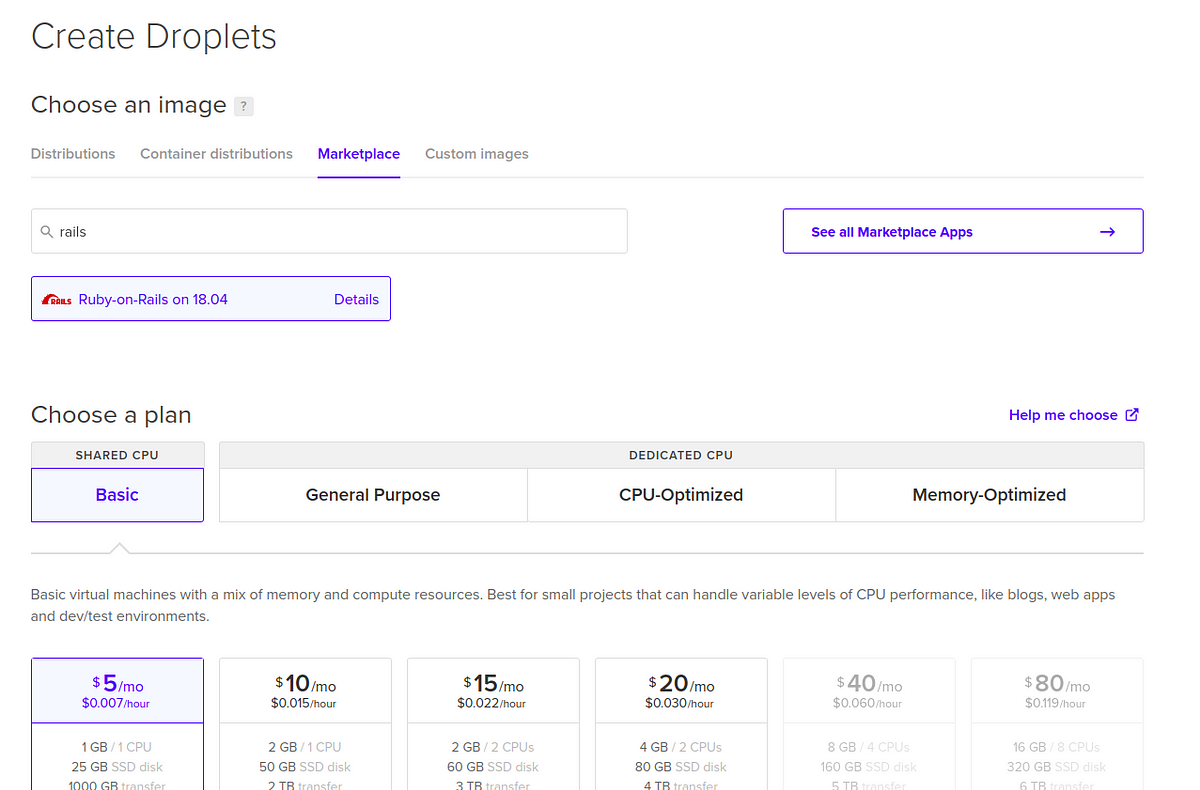This image is a screenshot from a website interface for creating droplets. At the top, the title "Create Droplets" is prominently displayed. Below it, the instruction "Choose an Image" is positioned, followed by a help icon represented by a question mark. The interface is divided into four distinct sections labeled "Distributions," "Container Distributions," "Marketplace," and "Custom Images."

The user has entered a search query for "rails," and the result shown is "Ruby on Rails on 18.04," written in a purplish hue, with a link labeled "Details" adjacent to it, also highlighted in purple. In the upper right-hand corner of the screenshot, there's a clickable text "See our Marketplace Apps," accompanied by an arrow, both in purple.

Further down the interface, under the "Choose a Plan" section, options are listed starting with "Basic," highlighted in purple. Other plan choices include "Dedicated CPU," split into "General Purpose," "CPU Optimized," and "Memory Optimized." At the bottom, different pricing options are visible. The pricing starts at $5 per month for 1 GB memory, 25 GB storage, and 1000 GB transfer. The next tiers are $10, $15, $20, $40, and $80 per month, each offering progressively higher resources.